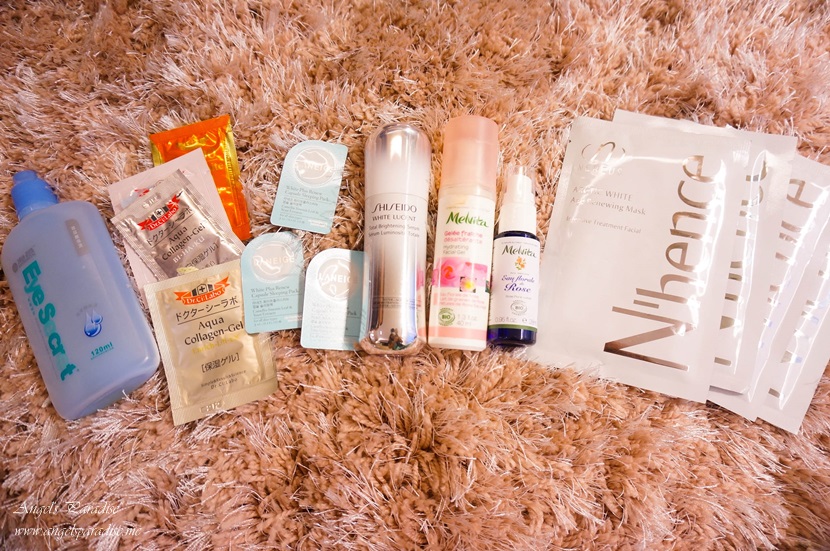This indoor photograph showcases an assortment of beauty products meticulously arranged on a brown rug background. Starting from the left, there is a blue bottle with greenish lettering that appears to spell "I, Scrose iSecret." Adjacent to this bottle are three white packets adorned with oriental lettering and a black line emphasizing "aqua collagen gel." Next, there are three small containers that resemble either contact lens cases or pill pouches.

Further to the right, a silver container with unreadable black text sits beside a white bottle labeled "Maluca" in green letters, featuring a peach-colored cap. A glass spray bottle, also labeled "Maluca," accompanies this arrangement. Concluding the display are four large white pouches with silver lettering that seemingly spell "N'hence." Each item's placement against the soft, textured rug enhances the detailed composition of the image.